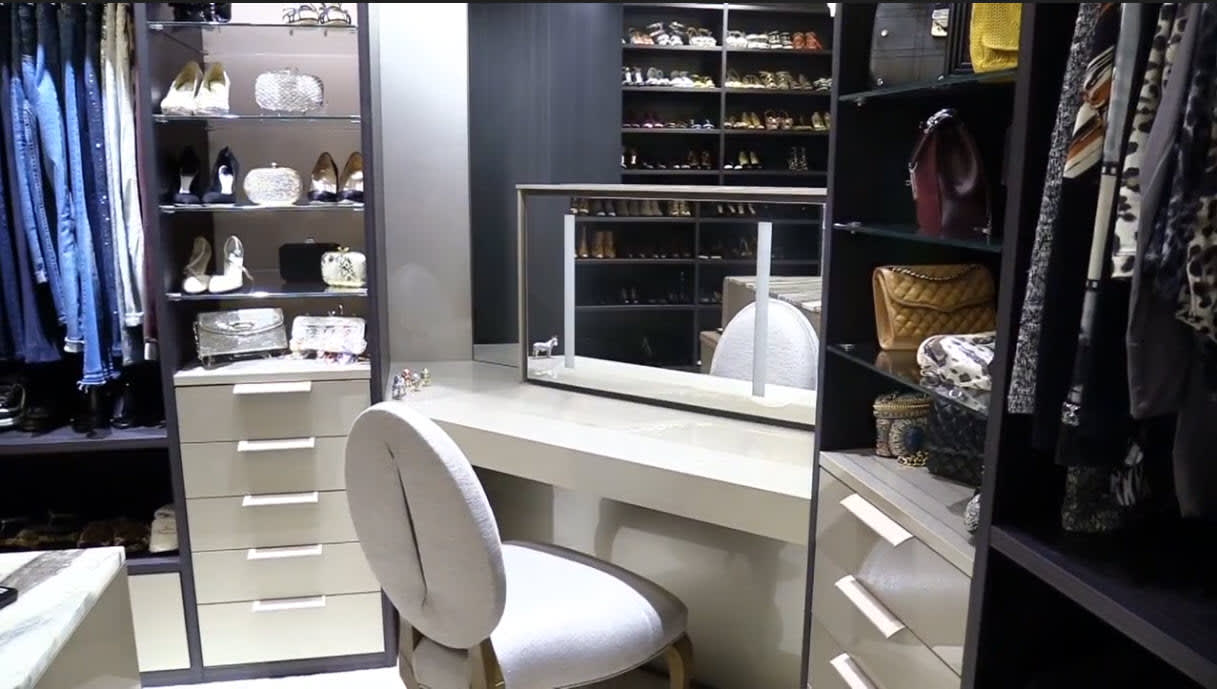This is a photograph of an elegant and meticulously organized walk-in closet or dressing room. At the center, there is a crisp white chair positioned before a white stone vanity table, which is paired with two mirrors: a closer, lower mirror likely intended for makeup application, and a secondary mirror behind it that offers a view of the room. The ambiance exudes sophistication and cleanliness. 

To the right of the vanity area, there is a black bookcase and wardrobe space. The wardrobe is neatly stocked with various women's clothing, including blouses and jackets, while the glass shelves prominently display an array of high-class bags and clutches. Further to the right, another section of the wardrobe features drawers and additional hanging spaces for more clothing items.

On the left side of the vanity, there are bookcases with glass display shelves showcasing an impressive collection of high-heeled shoes in diverse colors like black, white, and silver. Adjacent to this, there's a dedicated section for men's apparel, including blue and white dress shirts and a variety of shoes.

The overall setting is characterized by a stylish black-and-white color scheme, which further enhances the luxurious feel of this high-class dressing area.